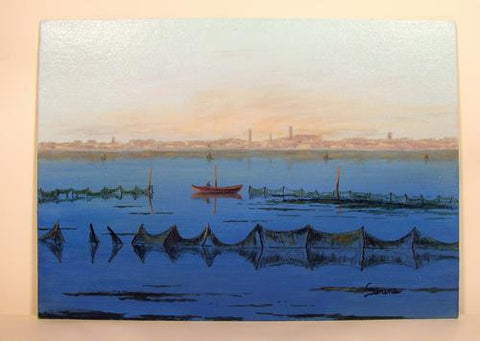This detailed painting, potentially an impressionist piece on canvas, captures a serene moment on a tranquil lake during the delicate magic hour of sunrise or sunset. Bathed in soft, orange light, the sky above merges into a light blue hue with faint, wispy clouds adorning the horizon. Central to this composition is a tiny, reddish-brown sailboat hosting a lone figure, calmly anchored amidst a placid expanse of dark blue water. Surrounding the boat are several long fishing nets, implied to be passively gathering fish. The far edge of the water meets a fuzzy, brownish backdrop suggesting an industrialized cityscape with tall smokestacks or the possibility of rows of homes, contributing an intricate depth to the scene. Despite the low resolution making fine details indistinct, the overall impression evokes a tranquil yet industrious moment frozen in time.